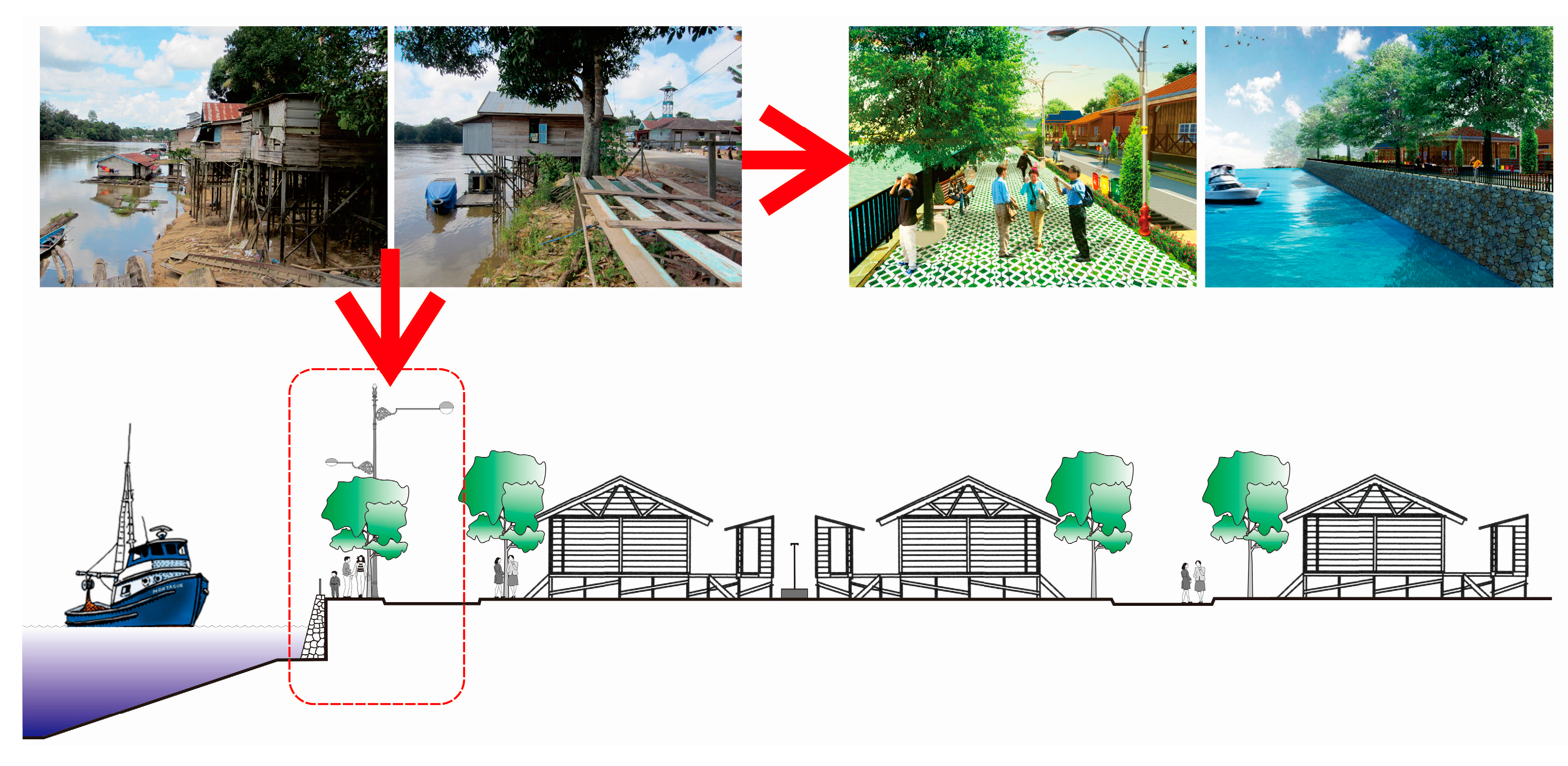This image is a detailed infographic set against a white background, depicting the transformation of a deteriorating waterfront area into a more developed, gentrified zone. In the top-left corner, there are two photographs of a dilapidated, low-income village with rundown shacks on a beach or watery area, and an overturned boat nearby. A red arrow points from these images to the right, indicating a proposed transformation shown in two more images. These mock-ups illustrate a revitalized waterfront: one depicts three business people standing by a large tree, next to a checkered sidewalk and a building, while the other shows a canal or river wall with a boat in the water, trees, and a building lining the right side. 

Below these images, another large red arrow points downward to a blueprint drawing. The blueprint details the proposed development steps and includes various elements such as a ship, a family standing under a tree with lampposts nearby, and a timeline-like sequence of different structures, alternating between trees and buildings. This layout highlights the envisioned transition from the current state of disrepair to a polished, organized waterfront community.